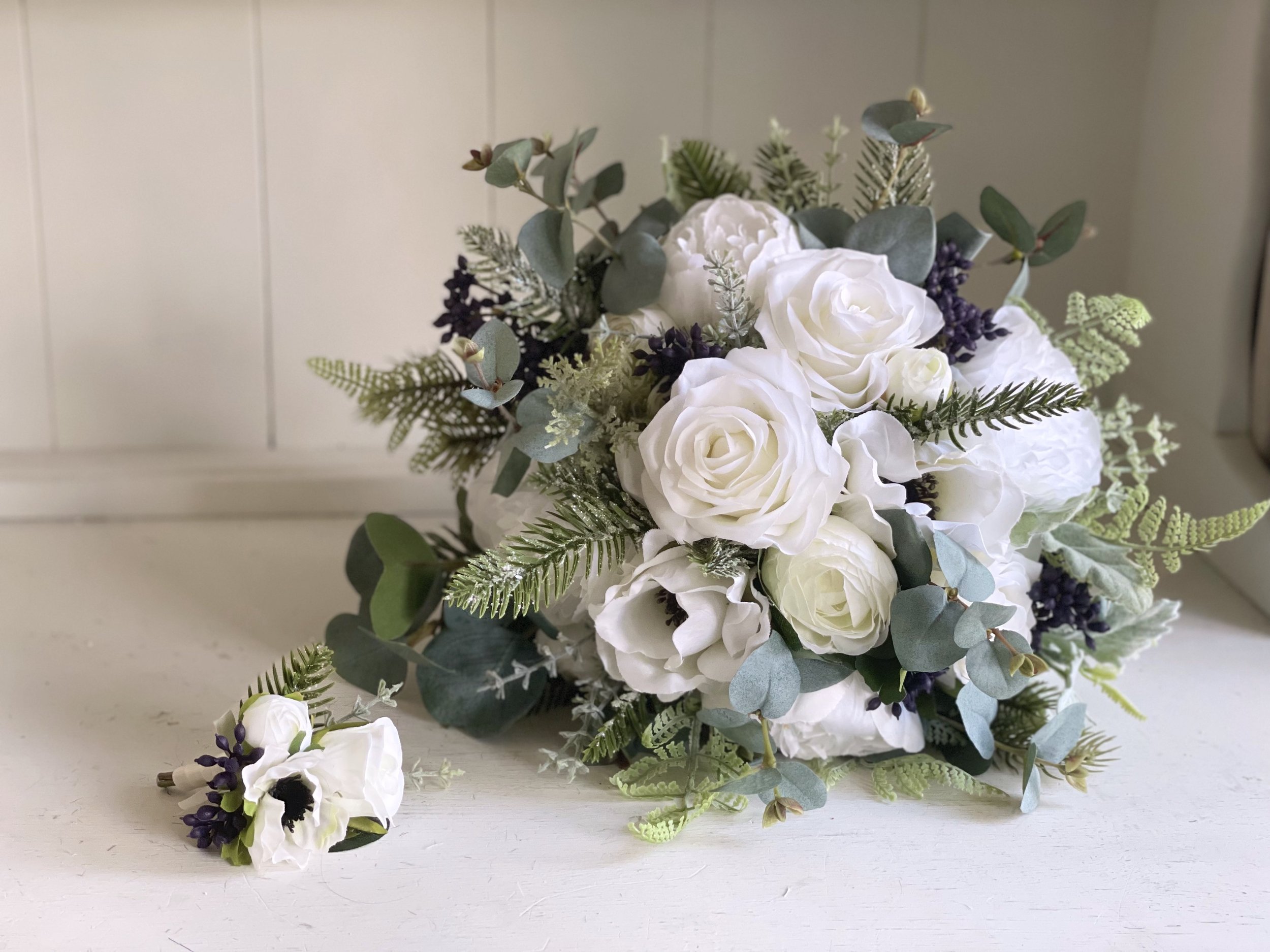The image is a landscape-oriented photograph featuring a meticulously arranged bouquet of flowers. Positioned just right of center, the bouquet rests on a pristine white surface, which aligns with a white wall adorned with vertical paneling and subtle light gray lines. The floral arrangement predominantly consists of white roses, accompanied by other white flowers and an array of greenery. The greenery varies in hue, displaying shades from light green to dark green, with some tinges of gray-green and blue-green. Interspersed among the foliage are small, dark blue buds or flowers, adding a delicate contrast to the ensemble. Adjacent to the bouquet lies a smaller boutonniere, also composed of a white rose with whitish greenery and matching dark blue buds. The striking combination of white flowers and diverse green tones suggests that the setup might be a wedding exhibit, showcasing a bridal bouquet and a groom's boutonniere against the minimalist backdrop of the white panelled wall.